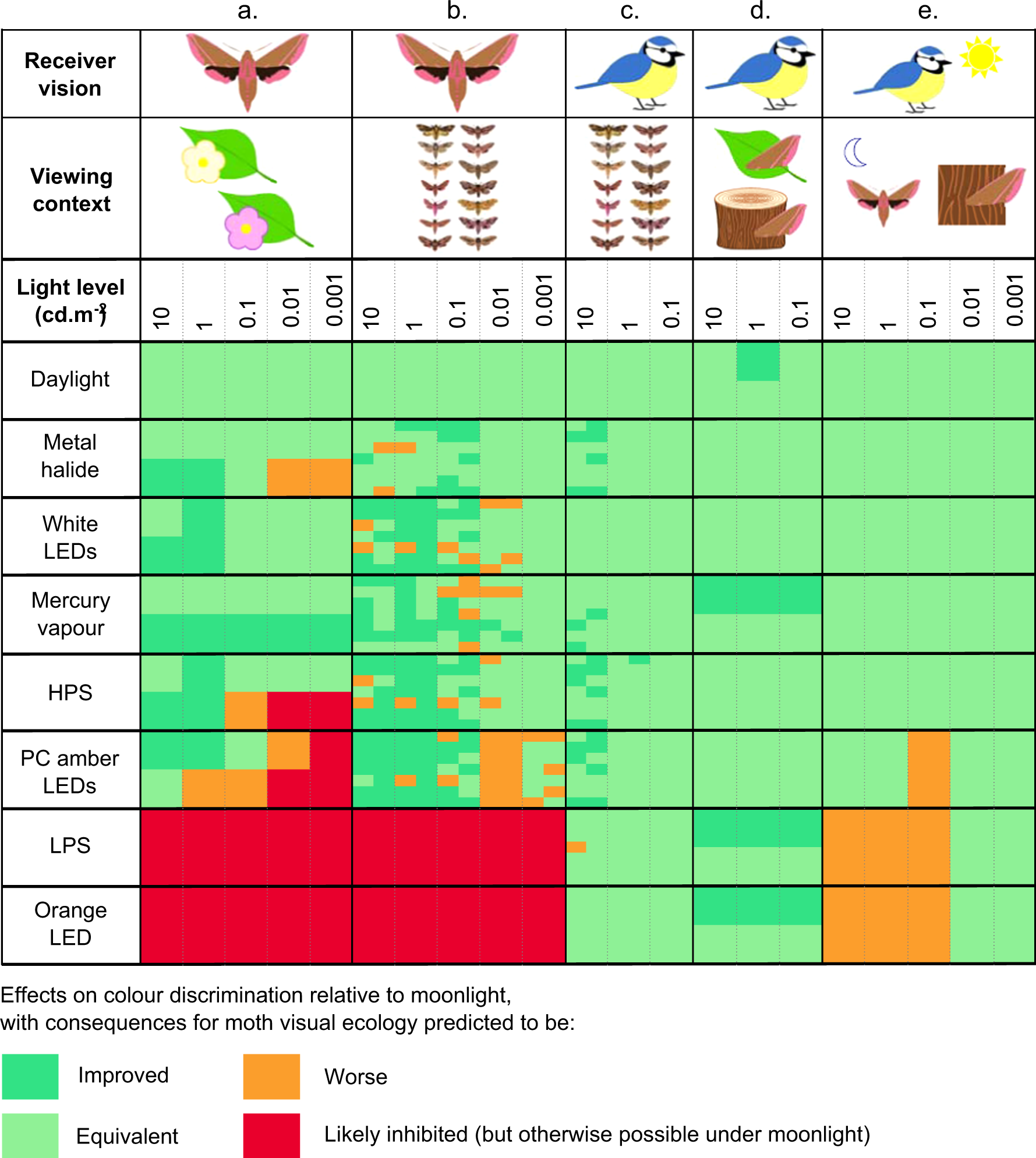The image is a detailed scientific graph related to ecology, specifically focusing on the visual ecology of moths and birds under various light conditions. The vertical rows categorize factors like "Receiver Vision," "Viewing Context," and various "Light Levels" that include daylight, metal halide, white LEDs, mercury vapor, HPS, PC amber LEDs, LPS, and orange LEDs. The horizontal columns show different species: two types of insects (likely dragonflies) under columns A and B, and three species of birds (bluebirds) under columns C, D, and E. The key at the bottom explains the color-coded effects on color discrimination relative to moonlight: dark green represents improved conditions, light green is equivalent, orange signifies worse conditions, and red indicates likely habitat inhibition but possible under moonlight. The graph projects the consequences for moth visual ecology under each light condition.